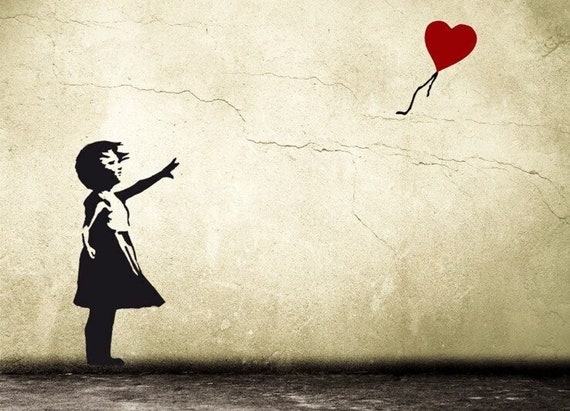The image depicts a widely recognized, simplistic mural painted on a cracked white wall. The mural shows a young girl, rendered in black and white silhouette, standing upright on a dark, gritty ground. Her hair and dress are swept forward as if blown by the wind. She extends her left arm towards a red heart-shaped balloon with a black string drifting away towards the top right-hand corner, symbolizing a poignant moment of letting go. Numerous cracks traverse the wall from left to right, adding to the mural's stark and weathered appearance.